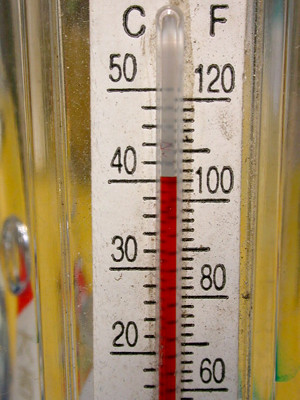The photo captures an outdoor thermometer with a white face, mounted in a clear plastic casing. The thermometer displays both Celsius and Fahrenheit scales on either side of a central mercury tube. On the left side, marked with a "C" for Celsius, the scale shows large numbers at intervals of 10 degrees, starting from 50 at the top and decreasing through 40, 30, and ending at 20, with smaller dashes marking each degree in between. On the right side, labeled "F" for Fahrenheit, the scale ranges from 120 degrees at the top, decreasing through 100, 80, and down to 60, also marked with smaller dashes between the larger intervals. The red mercury in the thermometer currently reads approximately 41 degrees Celsius. Behind the plastic casing is a yellow wall, suggesting the thermometer is mounted on an exterior surface.